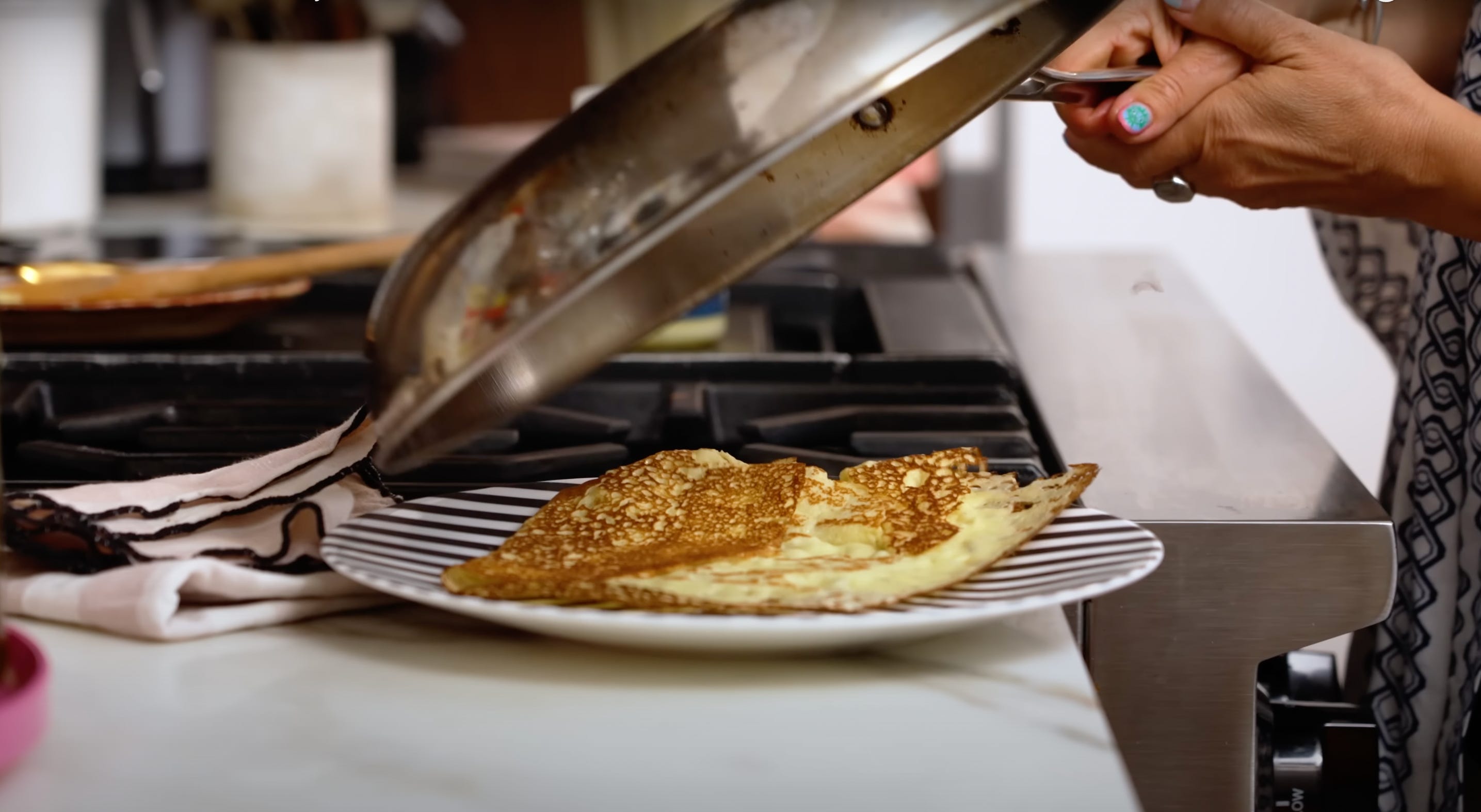The image depicts a kitchen scene where a person, identifiable only by their hands with teal nail polish, is in the midst of cooking. A crepe, already browned from frying, sits on a black and white striped plate positioned at the center bottom of the photograph. The person is seen holding a stainless steel pan above the plate, suggesting they have just transferred or are in the act of flipping the crepe onto the plate. Adjacent to the plate is a folded white dish towel. The backdrop features a gas stove with silver front and dark black grates, and a wooden spoon rests atop another pan on the stove. The overall setting includes a background element with utensils or other kitchen tools, though slightly blurred. The kitchen scene comes together with hints of additional equipment, such as a pink plate on the left edge of the image, emphasizing an active cooking environment.